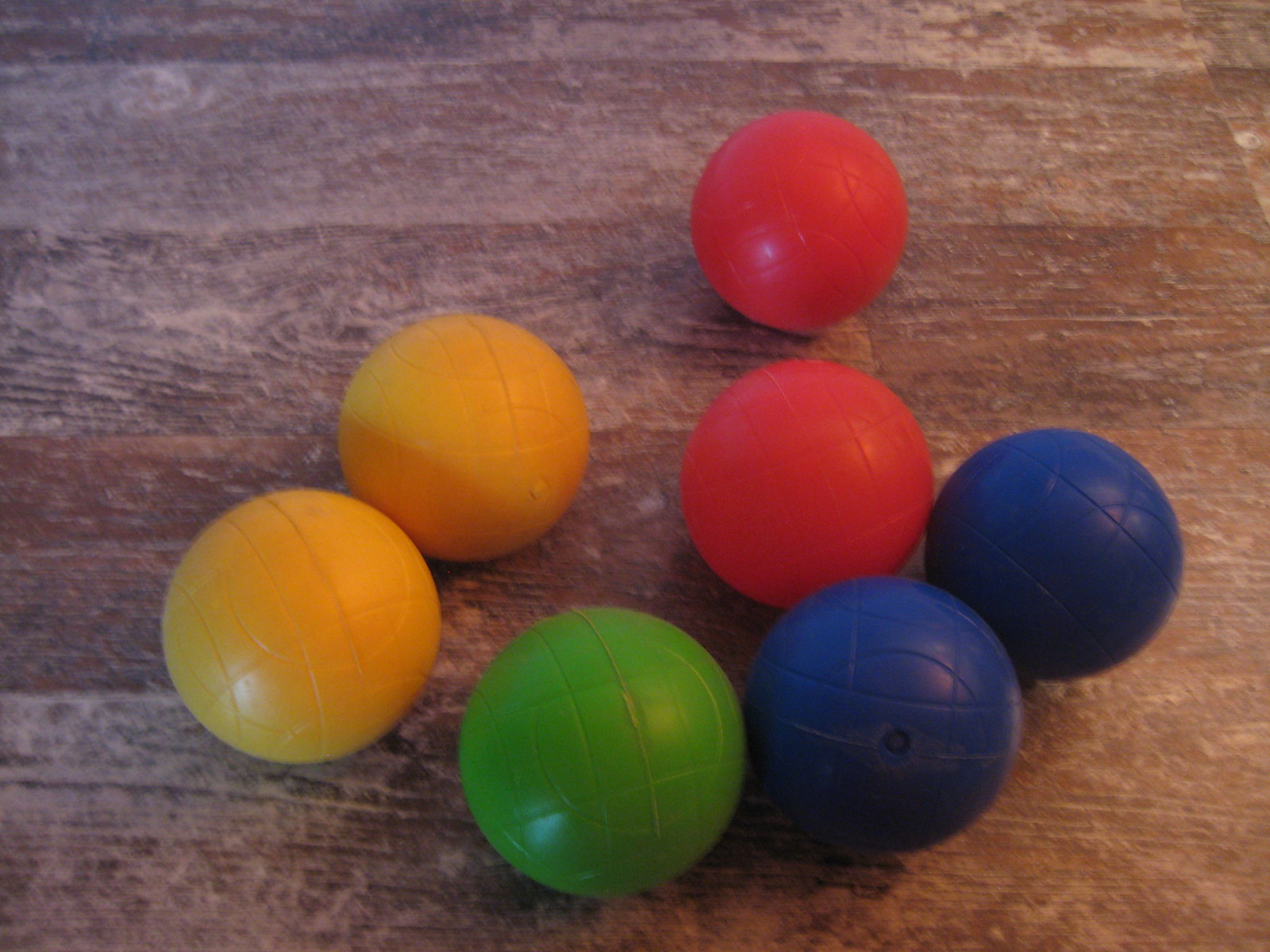The image depicts a scratched-up, light brown wooden floor of poor quality, with seven textured, foam-like stress balls scattered on the surface. The balls are patterned with lines and a circle in the middle, resembling mini soccer balls. 

The arrangement of the balls is as follows: two yellow balls are positioned together on the left side, followed by a green ball in the lower middle. Nearby, a blue ball is placed to the right of the green one. Above these, two red balls are aligned vertically, and another blue ball sits further right. Notably, one red ball is slightly distanced from the other six balls, which are otherwise grouped closely together.